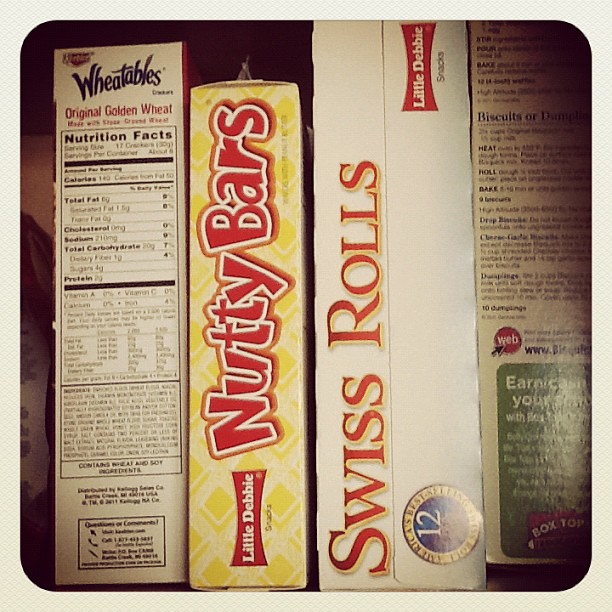The image depicts four food boxes standing upright side-by-side, possibly on a shelf within a pantry or cupboard. Starting from the left, the first box is Keebler Weedables, with "Weedables Original Golden Wheat" displayed in blue lettering and a nutrition label below. Moving to the right, the next box is Little Debbie Nutty Bars, featuring the Little Debbie logo vertically along the left side and "Nutty Bars" written in red letters with a white outline on a yellow hatched background. The third box is Little Debbie Swiss Rolls, predominantly white, with "Swiss Rolls" printed in red with yellow outlines, and the Little Debbie logo in the upper corner. The lower right corner of this box has a seal indicating “12.” The fourth and final box is a tan-colored box with some indistinct wording, possibly a recipe for biscuits. All boxes are aligned uniformly in a slightly dimly lit room.